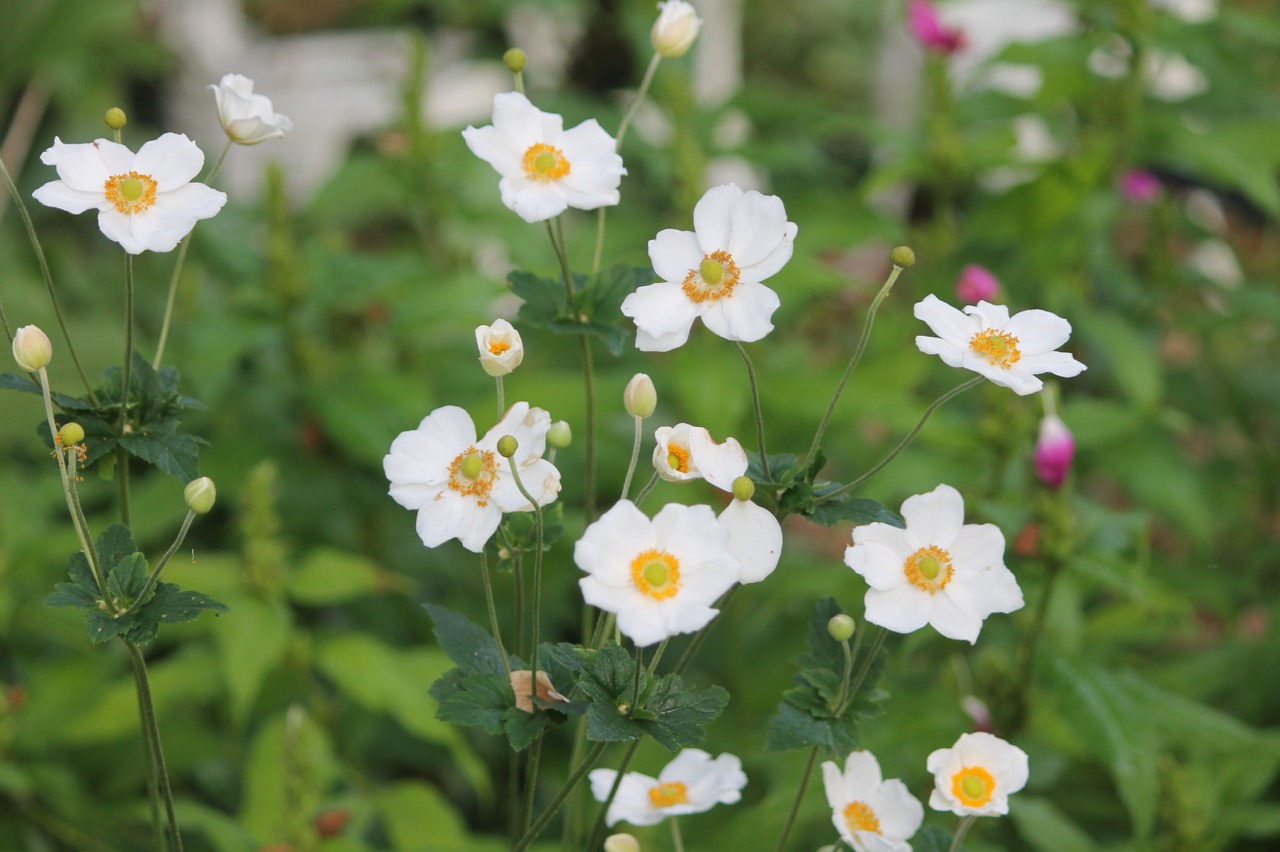This close-up photograph features a delightful cluster of white daisy-like flowers with six to eight petals each, radiating from vibrant yellow and green centers that have a subtle orange ring around them. These flowers, which give off a wildflower vibe, are showcased prominently on slender green stalks that rise from a base of lush green leaves. The flowers are in various stages of bloom—some are fully open, displaying their pristine white petals, while others are partially open or still in bud form.

The image's background is a beautifully blurred mixture of greens, suggesting a vibrant garden or field setting. Occasionally, hints of magenta and pink flowers add splashes of color to the otherwise green backdrop. A gray building and a tan or white chair are faintly visible in the distance, their details softened by the focus on the foreground flowers. The overall feel of the photograph is serene and picturesque, with an emphasis on the delicate beauty and varying stages of the white blossoms.